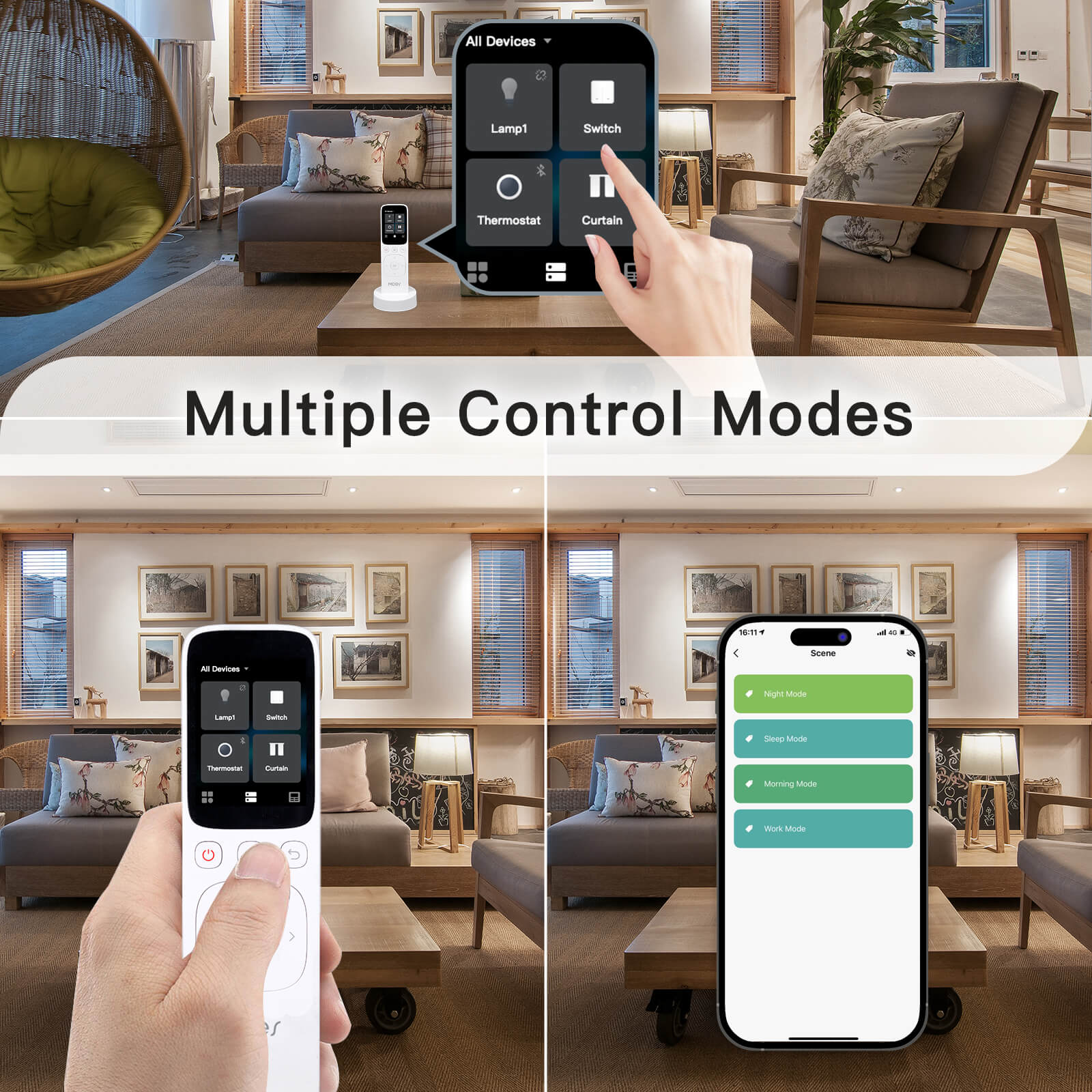The image is a vertical, digitally enhanced, full-color compilation displaying a living room scene with artificial lighting. The composition is divided into three main parts with thin vertical and horizontal lines crossing at the center. The top section features a Caucasian right hand interacting with a black display screen on a table situated in front of a brown couch and chairs. This display is of a full-sized white remote control in a stand showing various control options such as lamp, switch, thermostat, and curtain in speech bubbles. In the middle, bold black text within a white oval reads "Multiple Control Modes." The bottom half of the image presents two closer shots of the same room: on the left, a hand holds the white remote directly, using its buttons; on the right, a smartphone is used to control the devices, indicated by an app screen featuring alternating green and blue rectangles. The entire layout suggests multiple ways to manage home devices using either a traditional remote or a modern smartphone application, reinforced by the consistent living room decor across all sections.